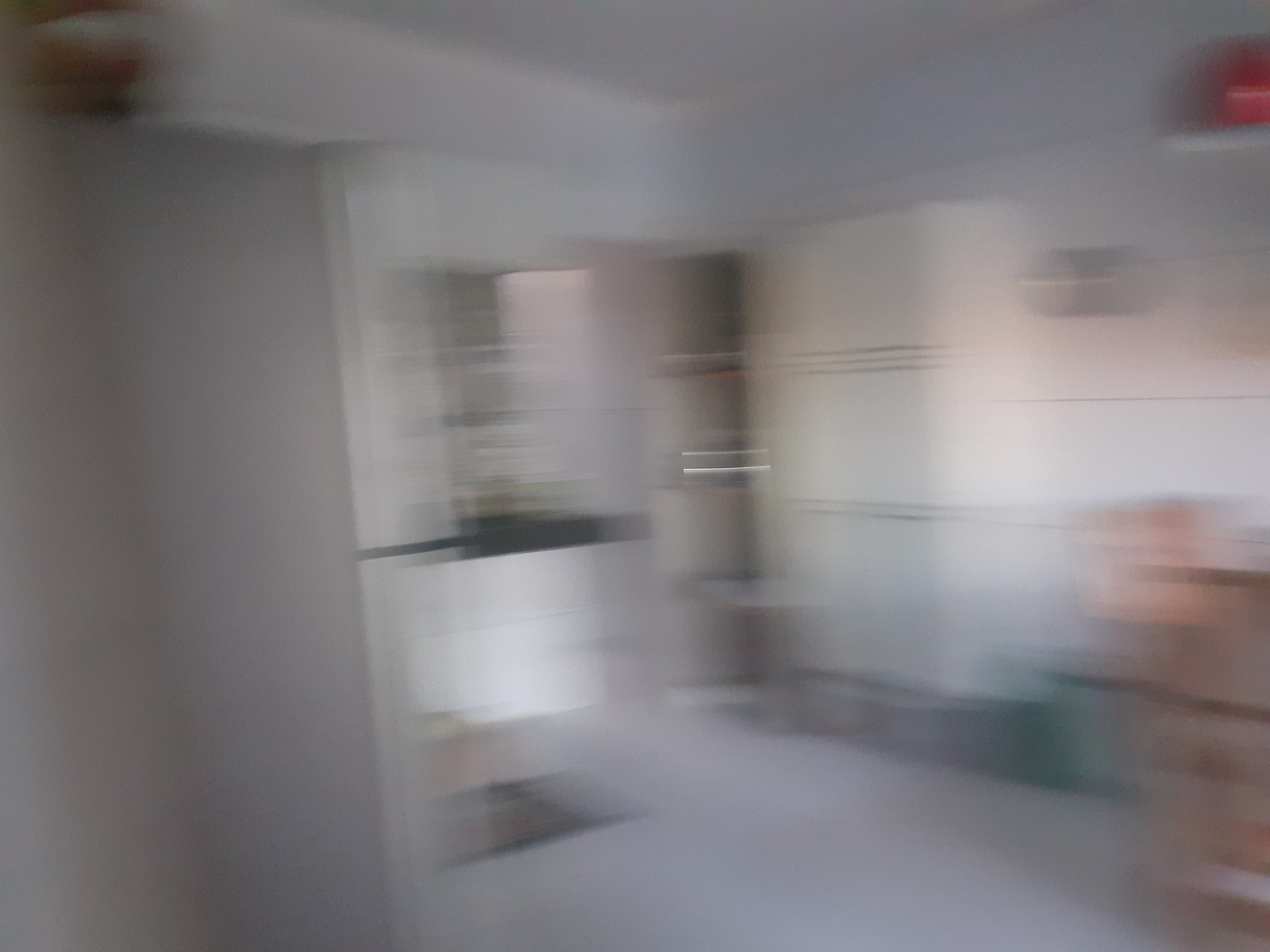This image captures the interior of a clinic, featuring a reception area with a sleek black countertop against pristine white walls. To the left (or right) of the counter, there's a closed shelving unit. Prominently visible are a green trash can, a fire alarm, and a wall clock. The clinic is furnished with a wooden table surrounded by reception chairs, and a floor mat adds a touch of comfort. Near the reception desk, recessed shelves are built into the wall. The room is brightly lit, enhanced by the white ceiling and linoleum flooring. The overall clarity of the image is somewhat compromised, giving it a slightly blurry appearance.